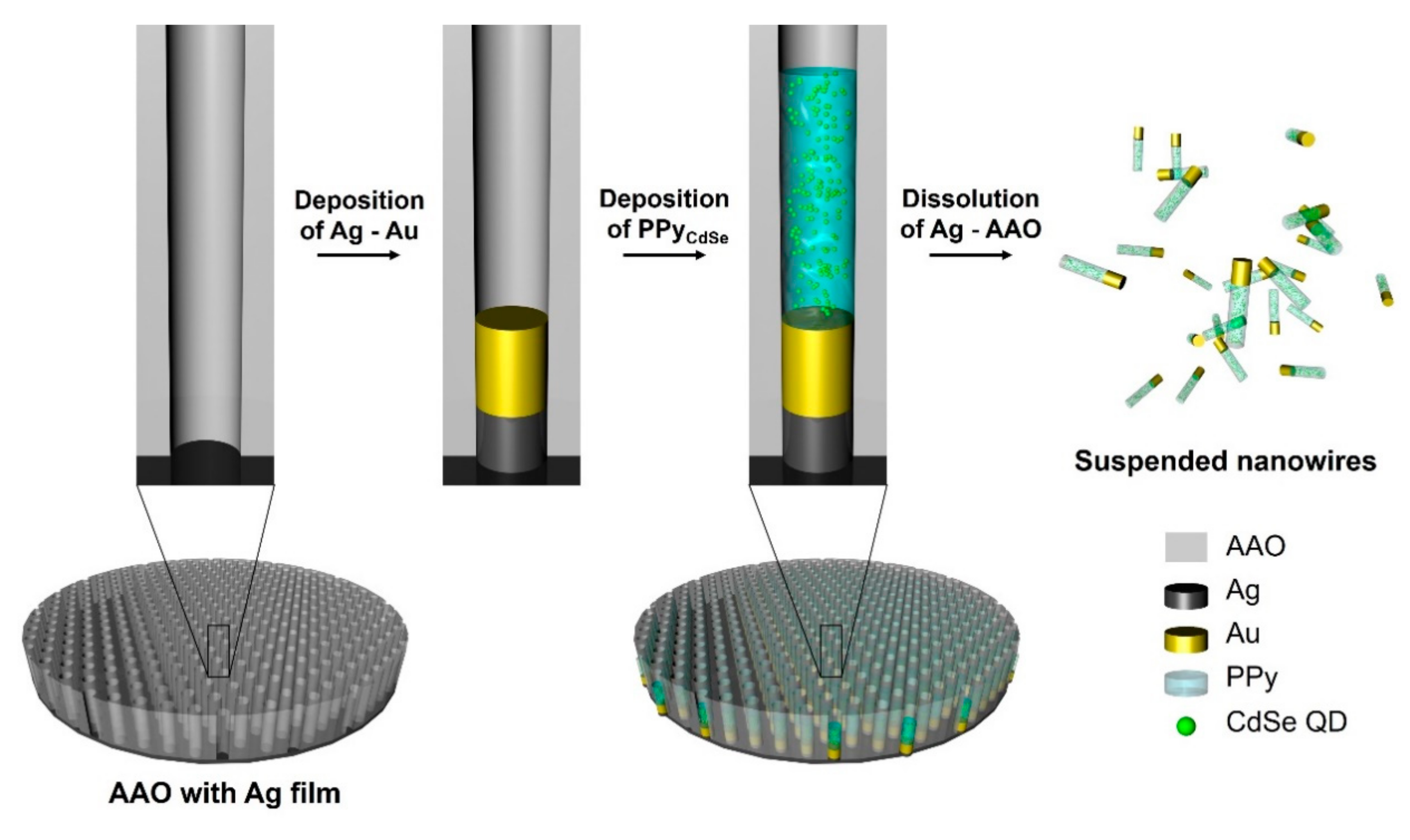The image is a textbook-like educational graphic with a white background, illustrating a sequence of chemical depositions and solutions within three tubes arranged horizontally at the top. The first tube, labeled "Deposition of AG to AU," is nearly empty, showing minimal liquid content. The second tube, labeled "Deposition of PPY-CDSE," contains a mix of grey and yellow liquids. The third tube, labeled "Solution of AG to AAO," features a complex mixture of grey, yellow, and blue-green liquids.

Each tube is connected by arrows, indicating a process flow from left to right. Below the tubes, the base of each tube is magnified and detailed. The first base, labeled "AAO with AG film," appears as a grey-colored circular image with spikes. The second base, associated with the second tube, shows a more detailed structure with distinct grey, yellow, and blue segments alongside green leaf-like structures.

On the far right of the image, there is a cluster of smaller, pill-shaped tubes containing yellow and green substances. Below this, black lettering reads "Suspended Nanowires AAO, AG, AU, PPY, and CDSE-QD," accompanied by a detailed key. This key clarifies that grey represents AAO, black symbolizes AG, yellow stands for AU, blue indicates PPY, and green denotes CDSE-QD, highlighting the varied components within the depicted nanowires.